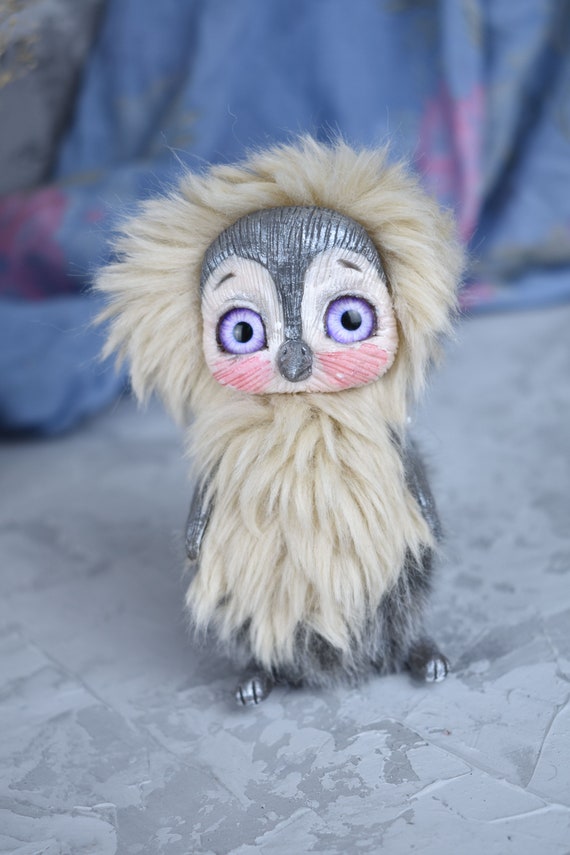The image is a color photograph of a handmade stuffed animal, resembling a fictional bird that merges features of an owl and a small penguin. The bird-like doll is positioned on a solid gray surface. Its face is predominantly white, accented with light pink highlights near its small beak, and features wide, light purple eyes with large black pupils. Rosy red cheeks add a touch of color to its face. The bird has fluffy, cream-colored fur on top of its head and around its chest, interspersed with white and beige hues. Beneath this layer, glimpses of gray and black feathers are visible, contributing to its whimsical appearance. It also has two arms and two small legs covered in similar tan fur. The background is slightly out of focus, revealing a draped blue cloth with pink and lighter tan designs.